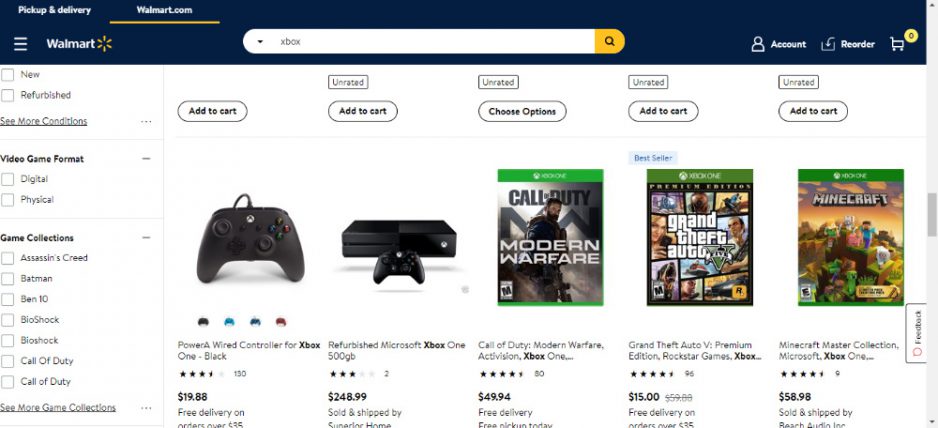The image showcases the Walmart website with its distinctive blue and yellow branding. At the top of the page, the prominent white Walmart logo is accompanied by its iconic yellow spark symbol. The blue header offers navigation options, including "Pickup & Delivery" and "Walmart.com," the latter of which is highlighted with a yellow underline. A hamburger menu with three lines appears, indicating additional options. 

Further down, a search bar with "Xbox select" typed in it takes center stage, accompanied by a yellow magnifying glass icon for initiating the search. To the right of the search bar, icons for "Account," "Reorder," and a shopping cart (which is currently empty) are visible.

Beneath the header, a row of navigational labels provides quick access to categories such as "New," "Refurbished," "See More Conditions," "Video Game Format" (digital or physical), and "Game Collections," which lists popular collections like Assassin's Creed, Batman, Ben 10, Bioshock, Call of Duty, and an option to "See More Game Collections." This section is set against a plain white background with black text.

The main content area prominently displays various Xbox-related products, including a sleek black Xbox controller and a refurbished Microsoft Xbox One console, along with their respective pricing and details. Featured games such as Call of Duty: Modern Warfare, Grand Theft Auto V Premium Edition, and Minecraft Master Collection for Microsoft Xbox One are also shown, complete with images and additional information.